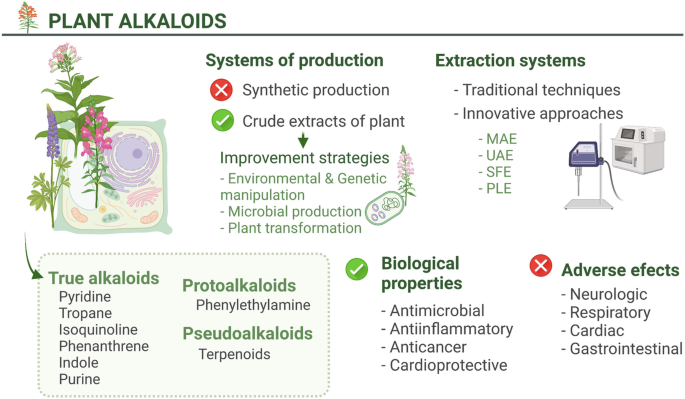The infographic titled "Plant Alkaloids" is prominently displayed in dark green at the top left corner, accompanied by a small stylized drawing of a green plant with yellowish flowers. This detailed technical sheet is divided into various sections, each thoroughly explaining different aspects of plant alkaloids.

Under the systems of production section, there's a red dot with an "X" marking synthetic production, and a green check mark highlighting crude extracts of plants. An arrow points downwards to improvement strategies, which are broken down into environmental and genetic manipulation, microbial production, and plant transformation.

The infographic thoroughly details different classes of alkaloids. True alkaloids include pyridine, tropane, isoquinoline, phenanthrene, indole, and purine. Protoalkaloids feature phenylethylamine, while pseudoalkaloids are represented by terpenoids. These categories are visually distinct with dark green headings and gray subtext, enclosed within a pale green rectangle bound by a dashed-dot border.

The extraction systems section lists both traditional techniques and innovative approaches, including abbreviated forms such as MAE, UAE, SFE, and PLE. An illustration of extraction machinery is depicted nearby, emphasizing the technical aspect of the process.

Finally, the biological properties of plant alkaloids are outlined, including antimicrobial, anti-inflammatory, anti-cancer, and cardioprotective effects. This is contrasted with potential adverse effects, which include neurologic, respiratory, cardiac, and gastrointestinal issues. Each of these points is presented with a green circle and white checkmark for benefits, and a red dot with a white "X" for adverse effects, reinforcing their seriousness. The entire infographic is presented on a white background with muted pastel illustrations, ensuring readability and aesthetic appeal.